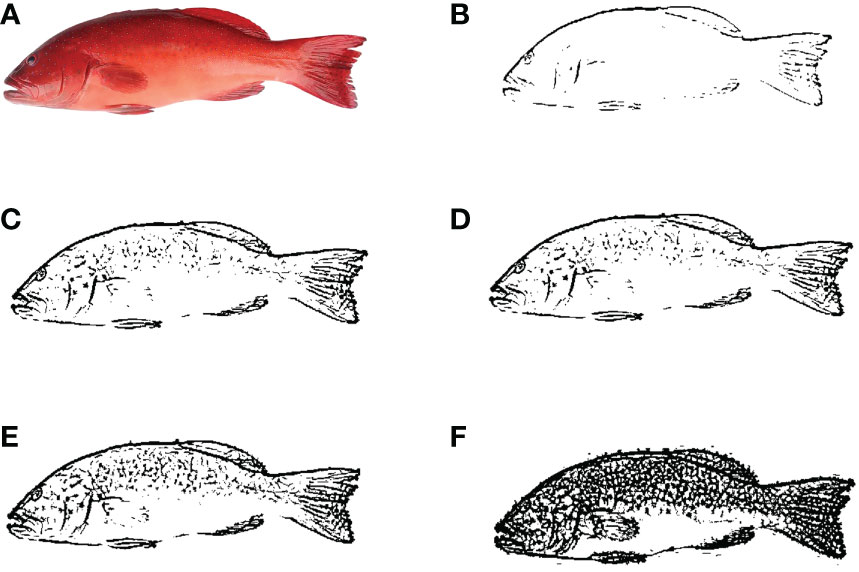This image functions as a detailed instructional poster on how to draw a fish, showcasing a step-by-step process through six stages labeled A through F. Starting with a full-color photograph of a red-orange fish under letter A (which is possibly a snapper or goldfish), the guide simplifies and evolves this image into a final black-and-white shaded drawing. Letter B begins with a basic outline of the fish. Moving to letter C, the outline adds more shading and details, albeit still monochromatic. In letter D, the drawing gains more intricate shading, which further refines the visibility of the fish's fins and overall form. Letter E continues this trend with more detailed shading, making the fish appear increasingly realistic. Finally, letter F culminates the process with extensive shading and texture, achieving a rich, detailed black-and-white illustration that closely resembles the original photograph.